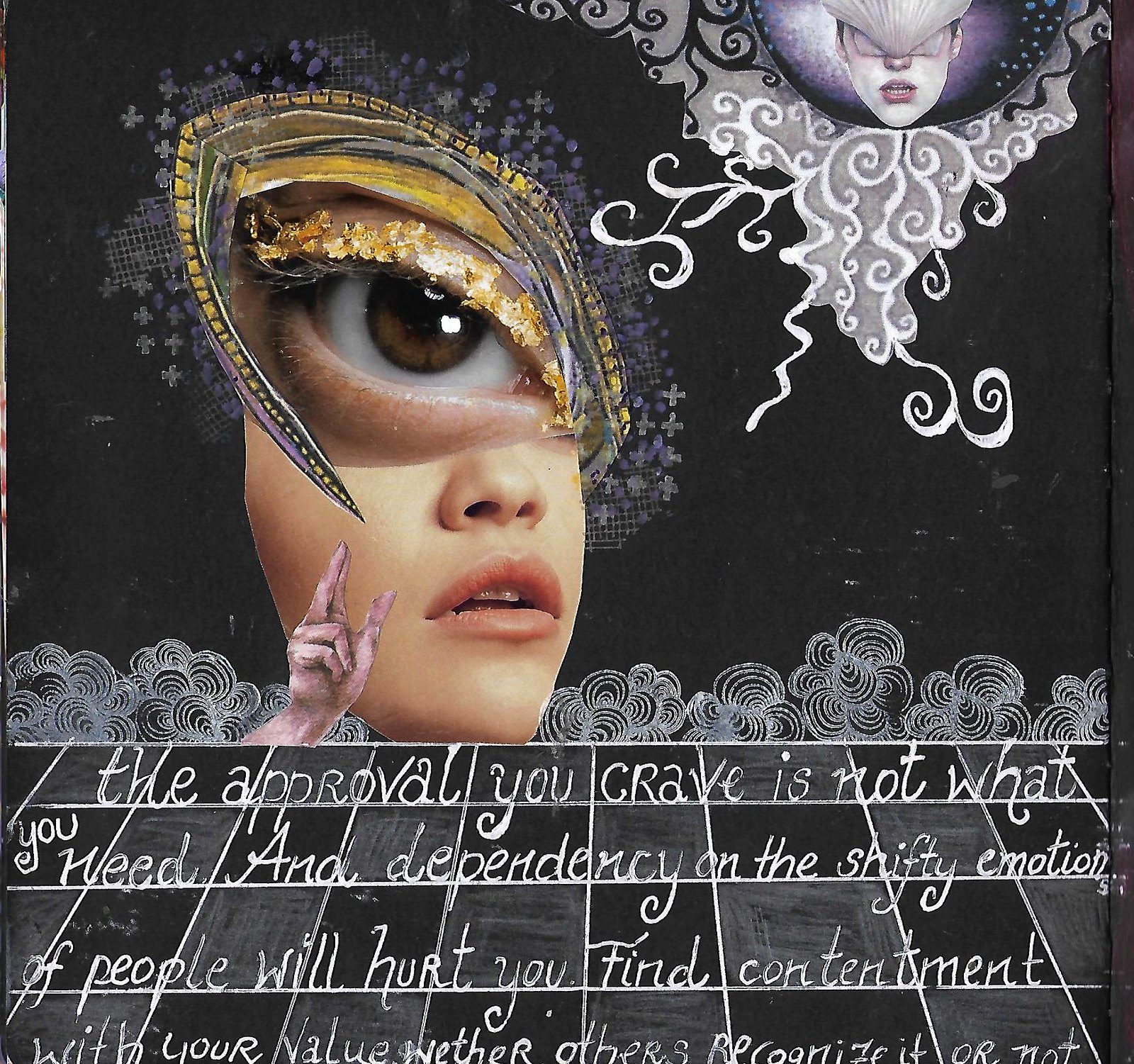This surrealistic art collage, set against a black background, features a mix of color photographs, illustrations, and typography in a square orientation. Dominating the top left is a partial profile of a woman's face from the nose to the chin, with a superimposed eye—complete with gold eyelashes and surrounded by stars—where the natural eye would be. Surrounding this eye, intricate golden illustrations add a layer of complexity. A hand is reaching up in front of this face, contributing to the collage's depth. To the top right, another woman's face is illustrated, with gray hair cascading over its eyes and enveloped in a gray circle adorned with stars and white scroll work. This intricate design extends downwards, framing the central elements.

The bottom portion of the image features a three-dimensional perspective checkerboard pattern, bordered with cloud-like motifs. Handwritten text across this checkerboard reads, "The approval you crave is not what you need, and dependency on the shifty emotions of people will hurt you. Find contentment with your value, whether others recognize it or not." This profound message is presented in white text, contrasting the black-and-gray checkered background, and accompanied by circular scroll work. The overall style fuses elements of collage, painting, and sketching to create a detailed and thought-provoking visual narrative.